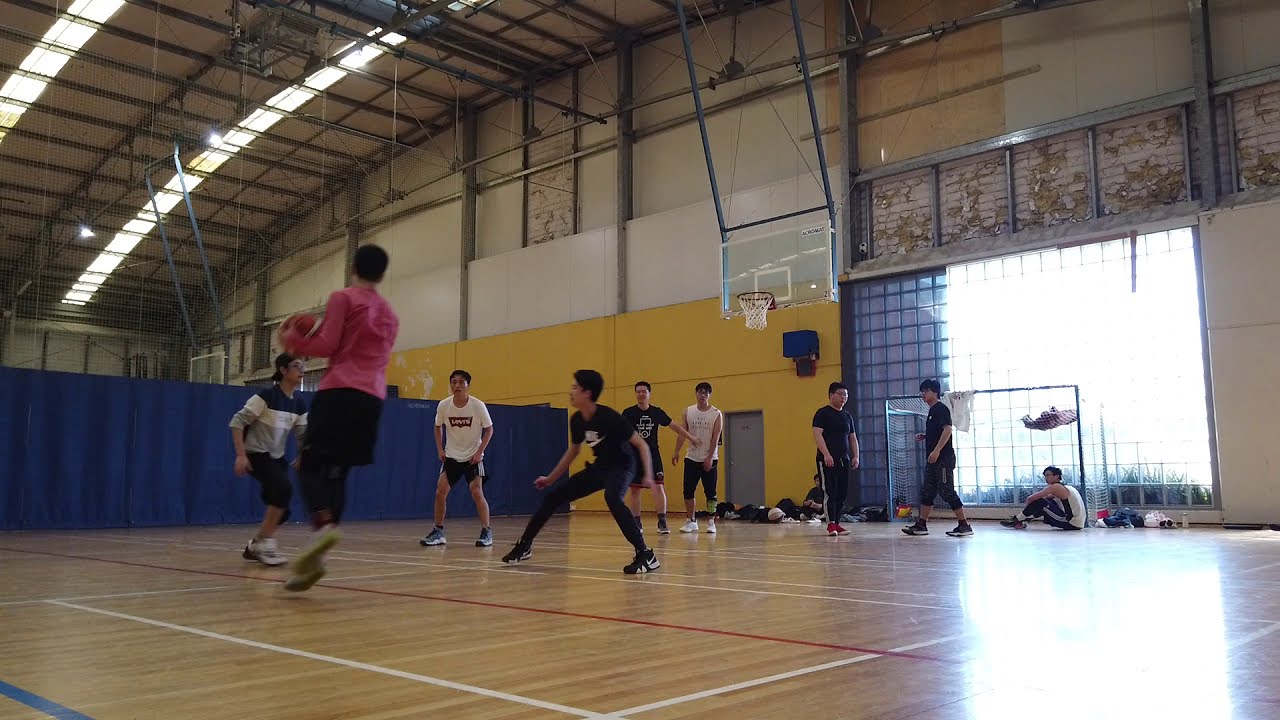In an expansive indoor gymnasium with tall ceilings and well-lit by overhead lights, a casual basketball game unfolds. This space, featuring a brown wooden court with painted white and red lines, is partially divided by a blue screen on the left, separating it into distinct sections. Prominent in the middle of the image is a basketball hoop with a glass backboard, suspended from the rafters by blue rods.

The action centers around eight high school-aged boys, possibly of Asian descent, identifiable by their athletic attire and the short black hair they each sport. The player closest to the camera, wearing a pink shirt and black shorts, is holding the basketball, his back to us as if preparing to pass. Surrounding him, to his left is a player in a multicolored shirt, to his right a boy in a white shirt, and directly beside him another in black shirt and black pants. Near the basket, two boys, one in a black shirt and the other in white, strive to block the shot, while just to their right another player in a black shirt and sweatpants faces off against an opponent in yet another black shirt.

Beyond the immediate action on the court, a seating area is discernible where a few spectators sit, framed by a large window with square glass panes that rise halfway up the yellow-painted walls. This image captures not only the dynamic movement of the players but also the ambient details—highlighting this practice session in a typical high school gymnasium.